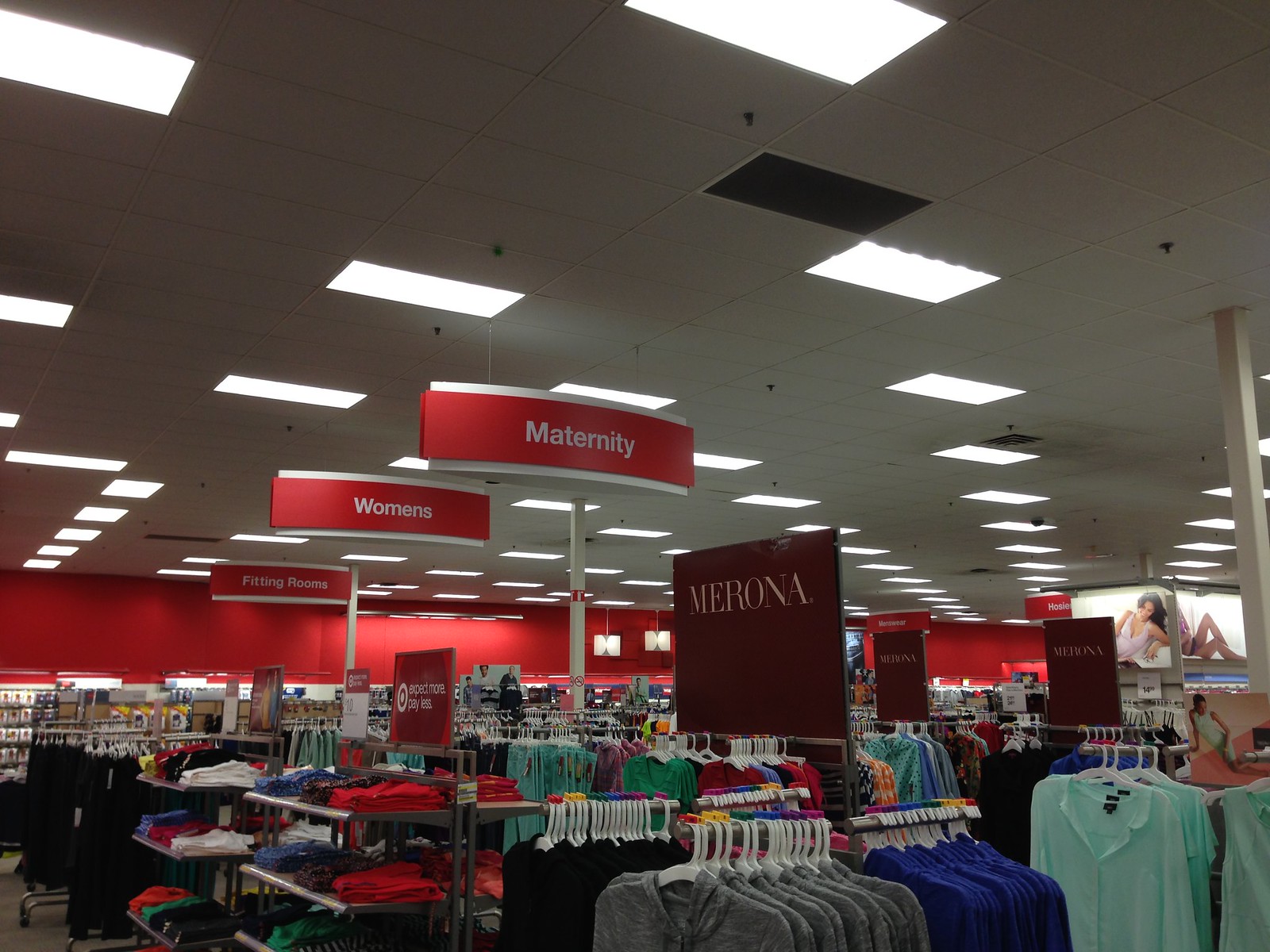This is an image taken inside the women's section of a Target store, showcasing a blend of vibrant colors and organized merchandise. Prominently featured in the center are three red signs with white text, each slightly curved at the edges and mounted on white poles. The first sign reads "maternity," followed by "women's," and "fitting rooms" further behind. In the background, red walls complement the signage, while the ceiling has a white drop design with fluorescent lights embedded in rectangular panels.

Beneath the signs and red strip, the space is filled with racks of women's clothing, displaying a variety of colors ranging from turquoise, blue, gray, and orange, to green, purple, salmon, striped patterns, periwinkle, black, white, and yellow. Glass shelves hold neatly folded tops. Additionally, there are Marona brand signs and images of female models in minimal clothing, enhancing the visual appeal and guiding shoppers through the selection. The ambiance is bright and inviting, emphasized by ample lighting and the orderly arrangement of merchandise.